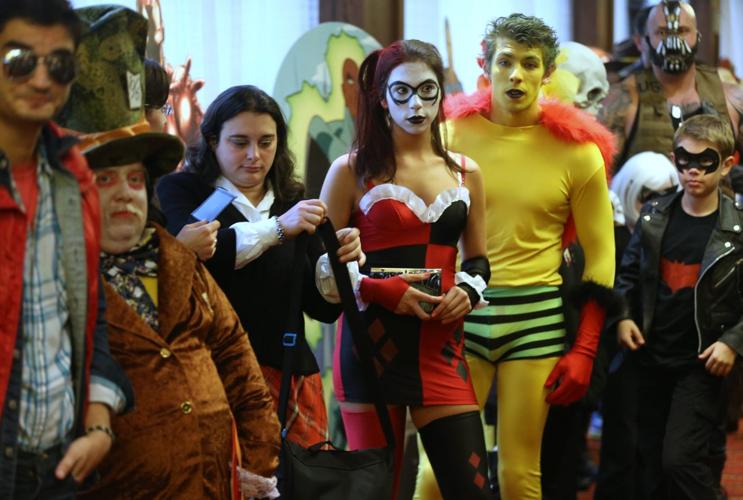In this horizontally aligned rectangular picture taken at a costume party, a vibrant group of eight to nine people are showcased, each adorned in unique and detailed outfits. The centerpiece features a woman with long, straight brown and red hair, painted white face with dark lipstick, and outlined black glasses that appear drawn on. She wears a spaghetti strap dress, black on one side and red on the other, adorned with card spades, paired with tall black stocking on her left leg and red stocking on her right.

Beside her is a man dressed in an eye-catching yellow outfit, accentuated by black and green striped shorts resembling underwear. He sports red gloves with black fur trim, a fluffy red cape, and has his face painted yellow with dark lipstick, complementing his short curly hair.

To the right, a young boy with short brown hair, dressed in a black leather jacket and painted mask, stands. His outfit includes a black shirt with a red bat logo.

On the left, a larger man in his 30s wears a tall hat with a green top and rim, an orange-circled face, a long brown velvet coat, and a large bow tie. Next to him, a woman in a black jacket, white shirt, red plaid skirt, and a black purse.

In the background, potentially a spooky skeleton head decoration adds to the festive atmosphere, with lacy curtains hanging on the windows of the room, further setting the scene for this lively costume party.